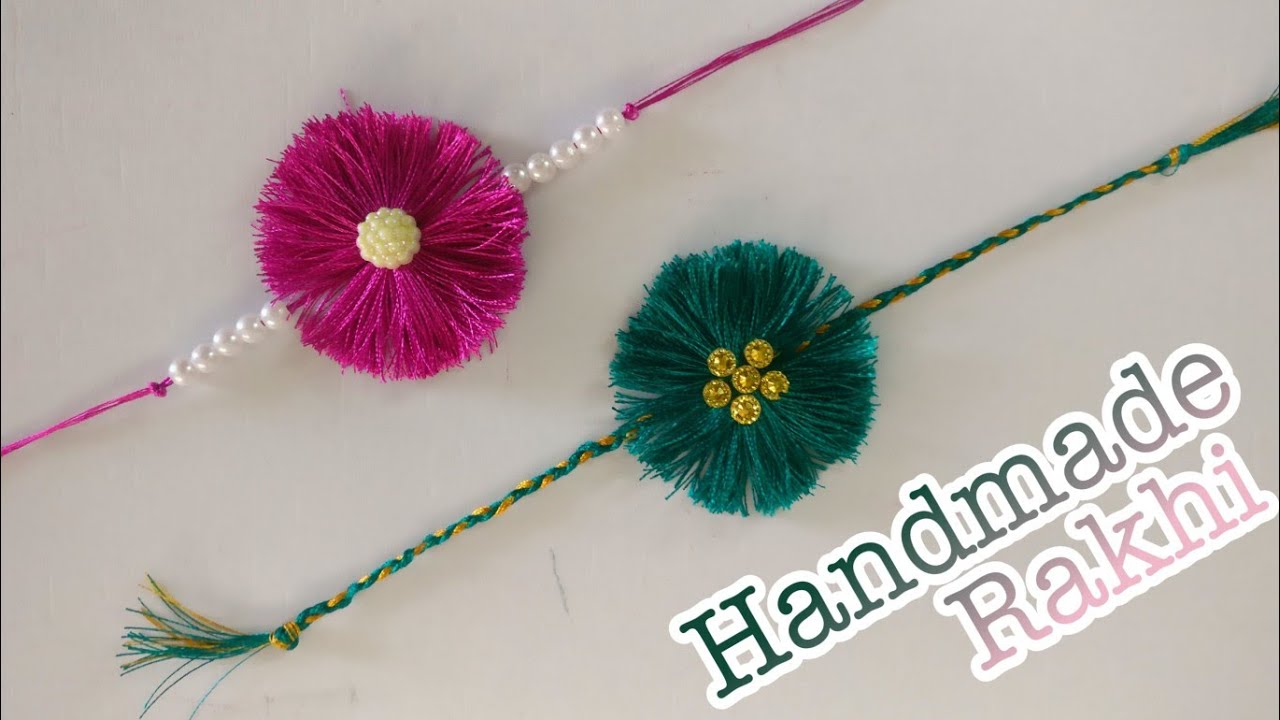This is a product image of two intricately designed handmade Rakhi bracelets, used in celebration. The background is a whitish gray with the words "handmade Rakhi" prominently displayed in black ink for "handmade" and a gradient of gray and pink for "Rakhi." The top bracelet is pink and features a stunning central flower made of circularly arranged pink strings. In the center of the flower, there is a stack of circular beads contributing a sense of depth and texture. On either side of the flower, five pearls are strung in a row leading to thinner strings. The bottom bracelet features a similar design with a green theme, having a braided string pattern. The center showcases a green flower with gold beads forming a five-point star at its heart, surrounded by more braided teal and gold strings. Both bracelets evoke the style of friendship bracelets and exhibit a handcrafted charm.